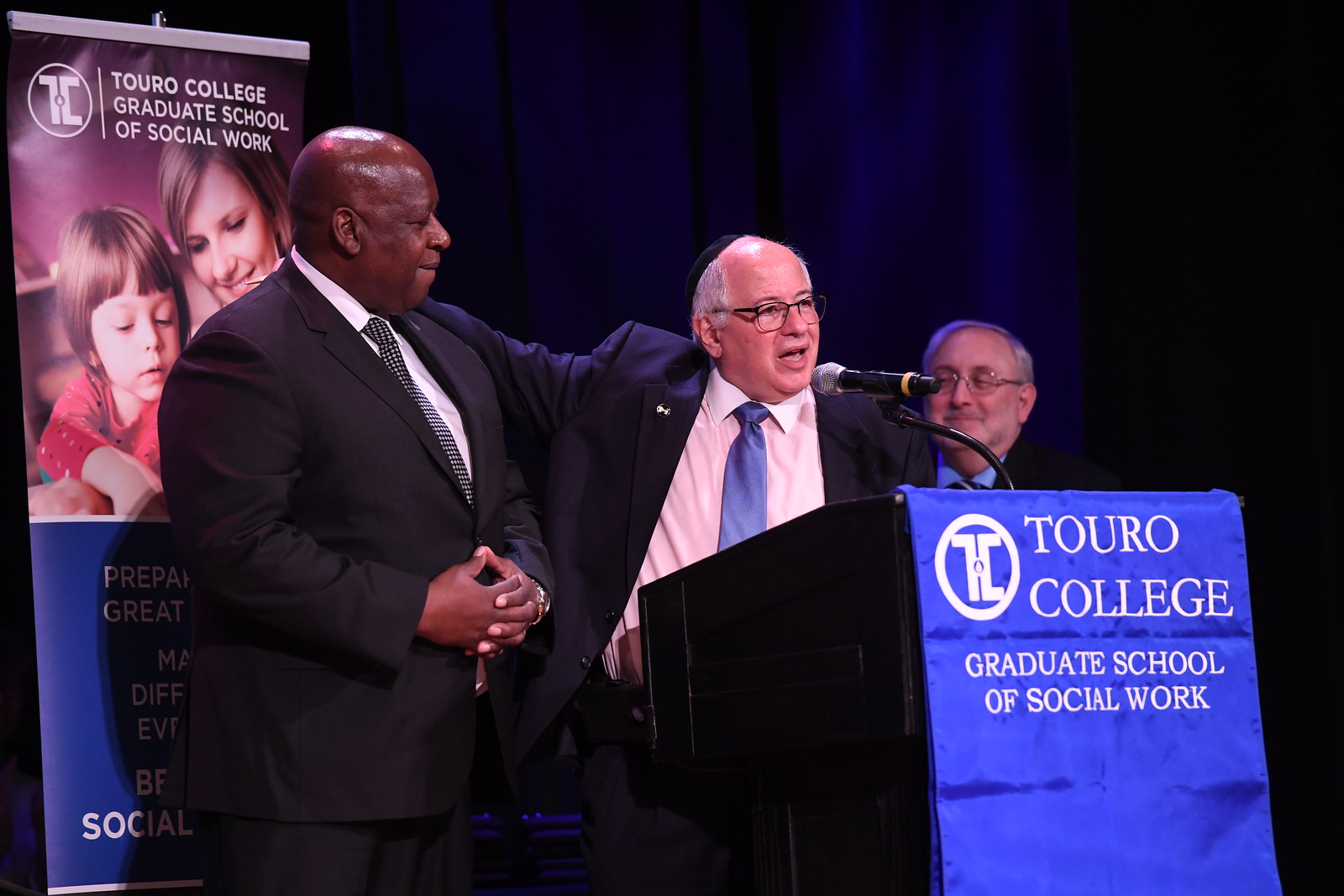The image depicts an indoor event at Touro College's Graduate School of Social Work, likely a commencement or an honoring ceremony. At the podium, a white gentleman with glasses and balding with gray hair on the sides is speaking into the microphone. He is wearing a blue tie and his right arm is draped over the shoulder of an African-American gentleman who stands to his left and appears to be the honoree. This African-American man is also distinguished by his stature and is dressed in a suit with a black tie patterned with white dots. His hands are clasped in front of him, and he looks content with the recognition he is receiving. Both men stand next to a lectern that prominently features a blue banner with the Touro College Graduate School of Social Work emblem, which includes a symbol of a 'T' and 'C' inside a white circle. In the background, a similar banner with an image of a woman and child further emphasizes the institutional affiliation and celebratory nature of the event. Another white man with gray hair is seen standing in the background, also in a suit. The overall scene is modern and solemn, fitting for a significant academic occasion.